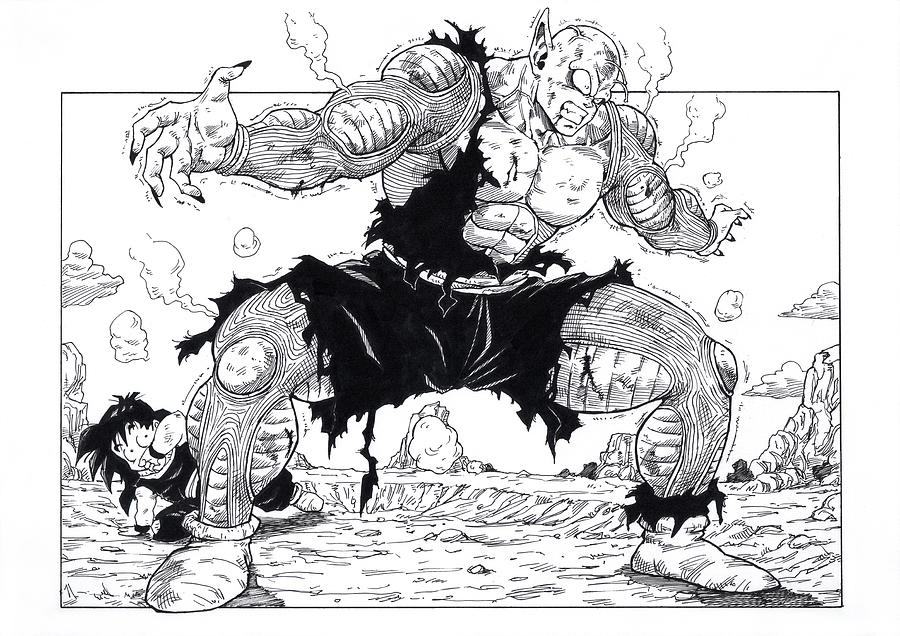This black-and-white illustration appears to be a scene from a Japanese manga or anime, reminiscent of Dragon Ball Z. At the center of the image is a colossal, muscular character with a goblin-like head, pointy ears, and a wide grin revealing his teeth. His bald head and small forehead are detailed with prominent veins across his body, emphasizing his immense strength. His clothes are in tatters, barely clinging to his bulging frame. Known as Vajada or a variation of that name, he is depicted going Super Saiyan.

In the bottom right corner, a much smaller character is captured in a moment of apparent fear, dressed entirely in black, with one hand covering his mouth. He is positioned slightly behind the towering figure, further accentuating the size disparity between them. The ground appears rocky, evoking a desert-like environment punctuated by a few scattered clouds in the sky. The smaller character's black hair and the contrast in sizes create a dramatic tension within this dynamic scene.